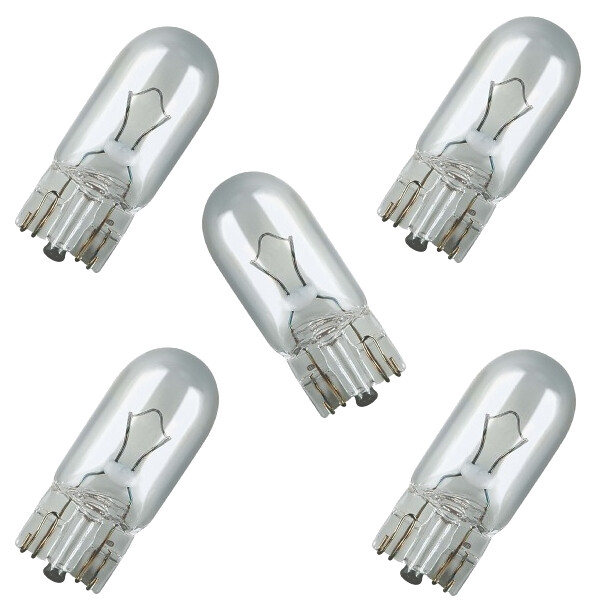The image shows five clear, oblong-shaped light bulbs with visible wire filaments inside. Each bulb has a flat, square-like base designed to slide into a specific socket rather than screw in, resembling automotive bulbs used in vehicles like tail lights. The bulbs are arranged with two pointing to the right and top, the middle one pointing to the left, and the bottom two pointing to the right. A distinctive white circular band encircles each bulb's middle, and a small round metal object is positioned beneath the plug-in section. These bulbs are clearly for specialized use, evidenced by their unique attachment system and clear, dome-shaped glass design that showcases the filaments.